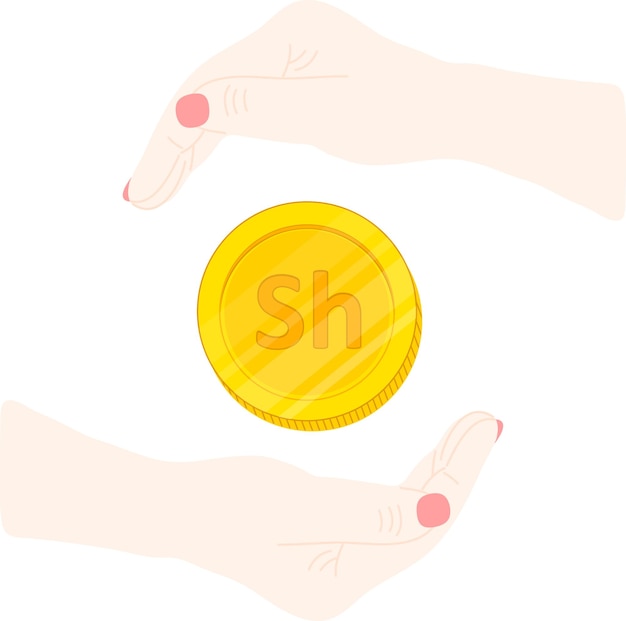The image depicts a computer-generated or cartoon-style artwork featuring two right hands cupping a coin-like object. Set against a vertical white rectangle background, the first hand emerges from the left and curves inward, with its painted pinkish-red thumb and index finger visible. The second hand, also from the left but positioned lower, has its palm upside-down, cupping the object from below. This object bears a resemblance to a checker or poker chip, rendered in a gold or yellow hue with slightly darker, ridge-like lines along its edge. At its center, the capital letters "S" and "H" are embossed with dark yellow, almost orange lettering. The overall composition of the hands and coin creates a three-dimensional effect, with hints of pink dots at the oblique sides of the coin.